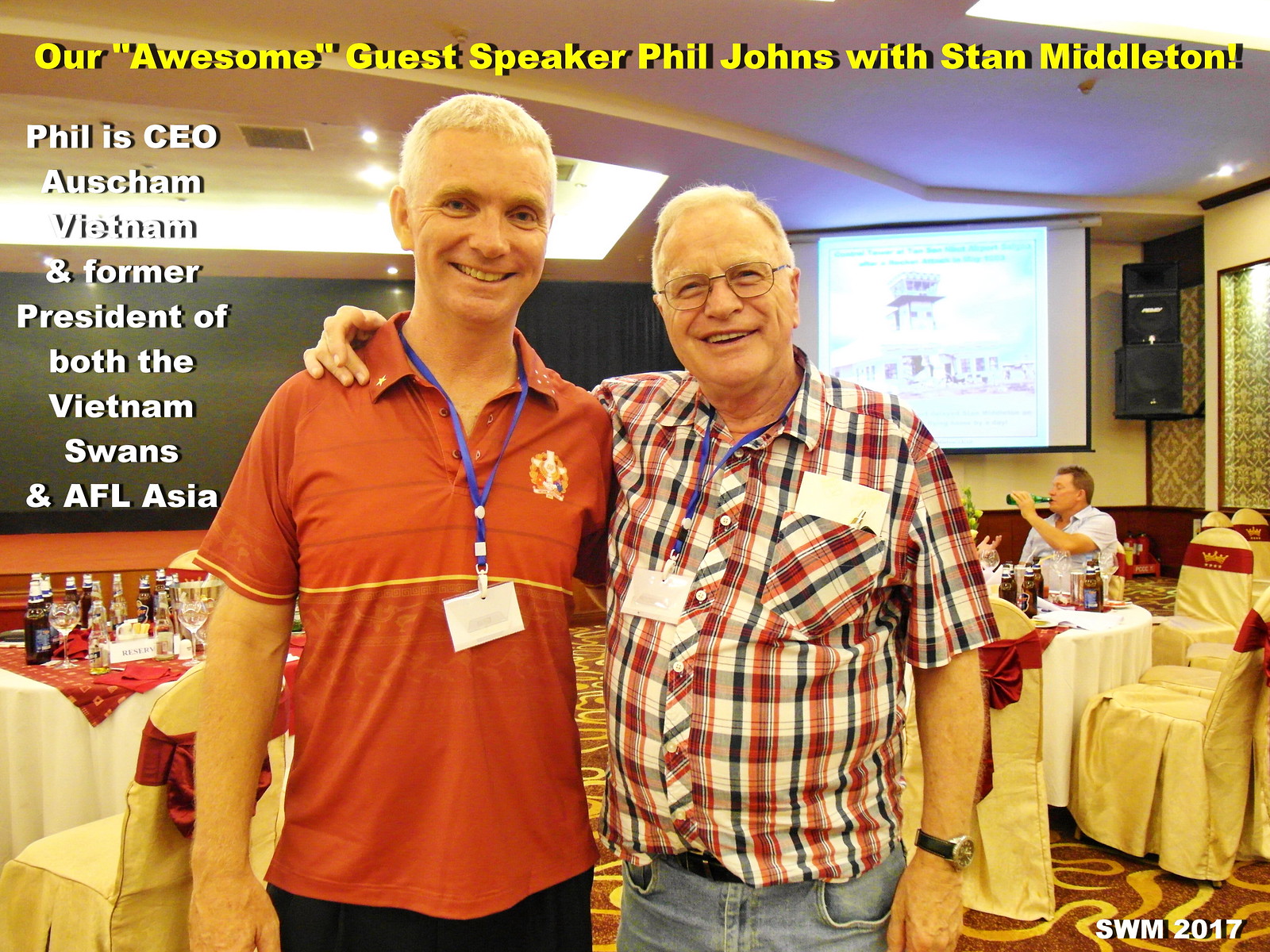In the photograph, two gray-haired men stand shoulder to shoulder, arms draped over each other in a friendly manner, in a hotel banquet lobby. The man on the left is wearing a red shirt and black pants, with a name tag around his neck. The man on the right sports a patterned red, blue, and white plaid button-shirt, with an envelope in the pocket, blue jeans, and a watch on his left wrist. Both men wear blue identification badges around their necks. Behind them, the hall is filled with tables adorned with white tablecloths and golden or cream-colored chair covers. These tables are scattered with numerous beer bottles. To the right, a large monitor displays a blurry image, surrounded by large speakers, and directly below, another man can be seen drinking from a beer bottle. Above, yellow text proclaims, "Our Awesome Guest Speaker, Phil Johnstown Middleton." To the left, additional vertical text reads, "Phil is CEO of AUSCHAM Vietnam and former president of both the Vietnam Swans and AFL Asia." The bottom right corner of the image features the text "SWM2017."